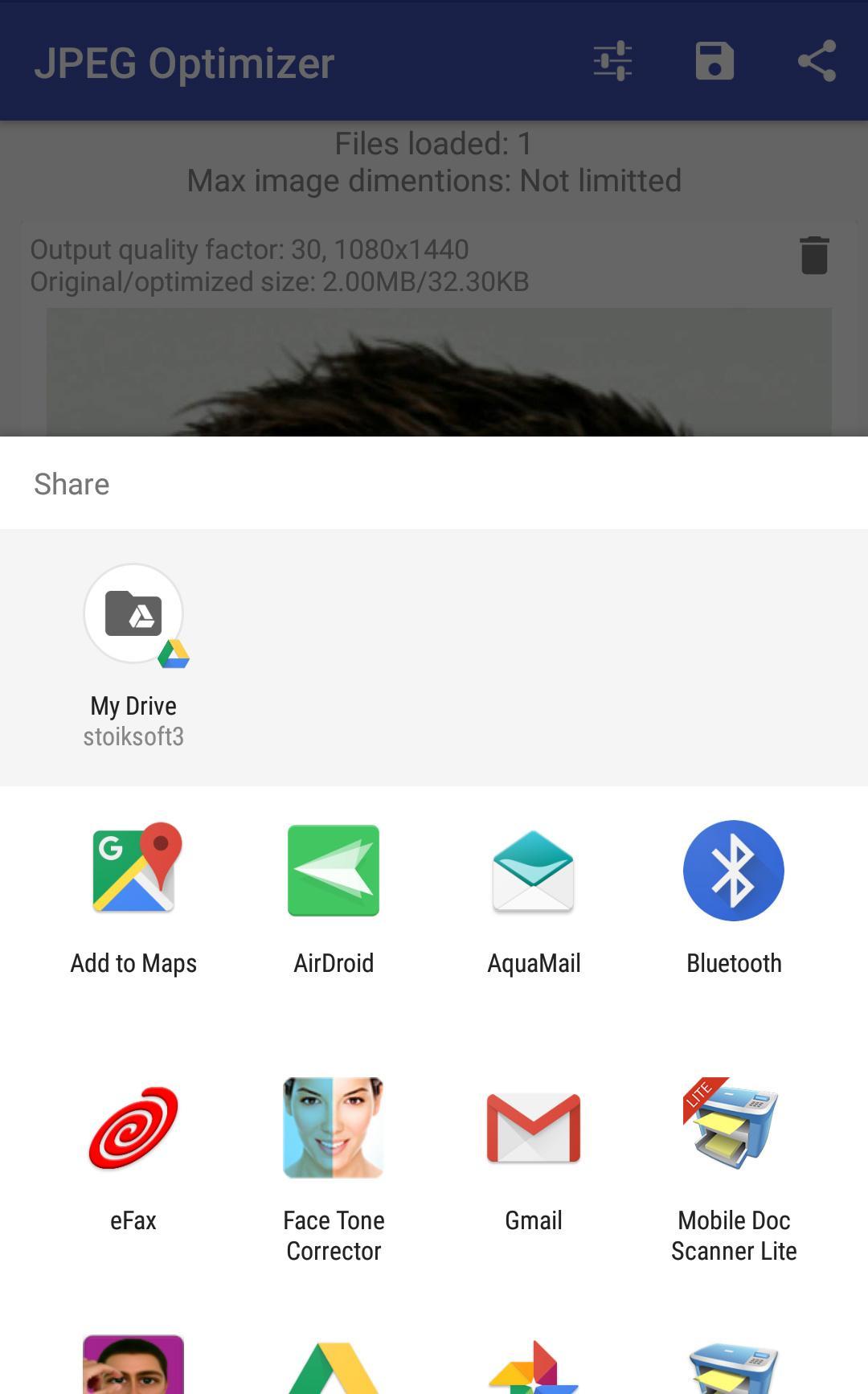The image displays a screenshot of a sharing interface within an app. At the top left corner, there's a "Share" button. Directly below it, there's an icon depicting a file, labeled "My Drive." The name "S-Toy K-Soft 3" is listed under this section. The screenshot also shows various app icons to which content can be shared, including Maps, AquaMail, Bluetooth, AirDroid, Gmail, FaceTone Corrector, eFax, and MobileDock Scanner Lite.